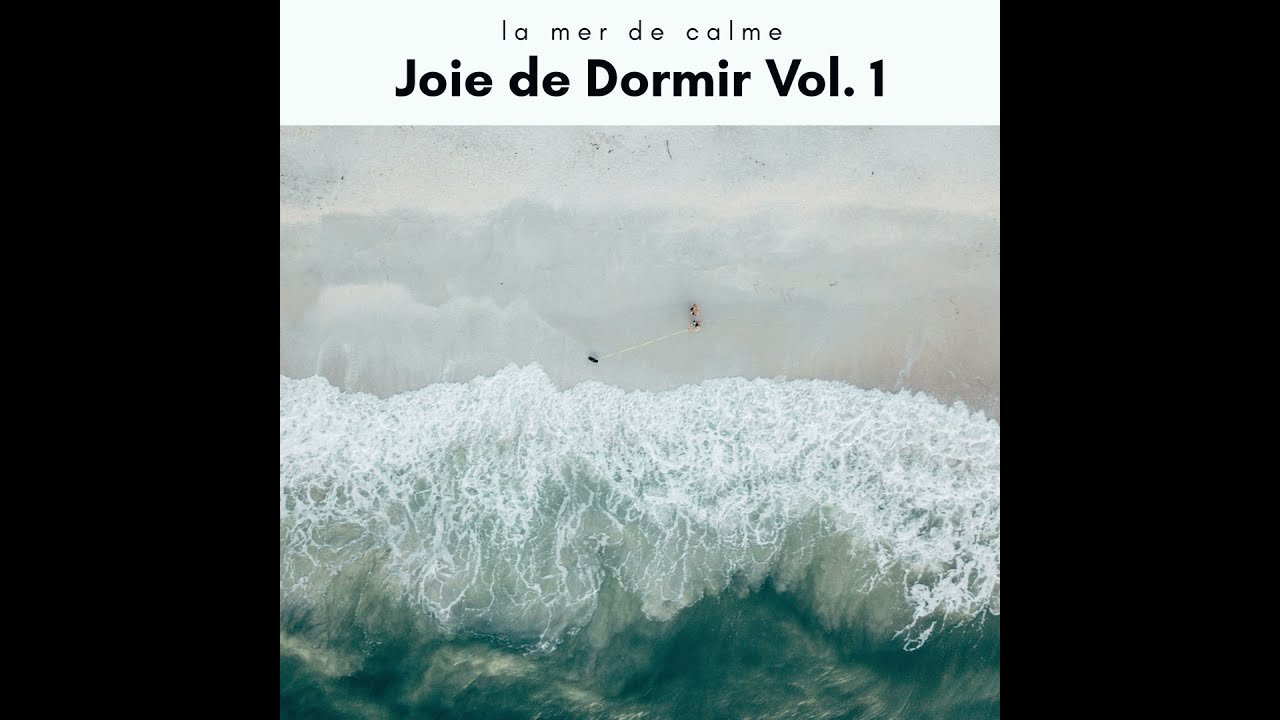The image seems to depict the cover of an album or art exhibit titled "La Mer des Combes, Joie de Dormir, Volume 1." Centered in the scene, and dominating the lower part of the composition, are white-capped waves with a mysterious, spongy texture reminiscent of soft moss against a bluish-green sea. The sky is a stormy gray, suggesting incoming or ongoing rain, and occupies the middle third of the image. The top third houses the text in a thick black font, with "Joie de Dormir Volume 1" prominently displayed and a smaller, thinner line of text reading "La Mer des Combes" above it. Borders of deep black frame the right quarter of the image and a corresponding vertical section on the left, while the central square holds the main visual elements. The overall colors are a palette of white, black, gray, and bluish-green, evoking a serene yet tumultuous seascape likely intended to suggest soothing ocean sounds for relaxation or sleep.